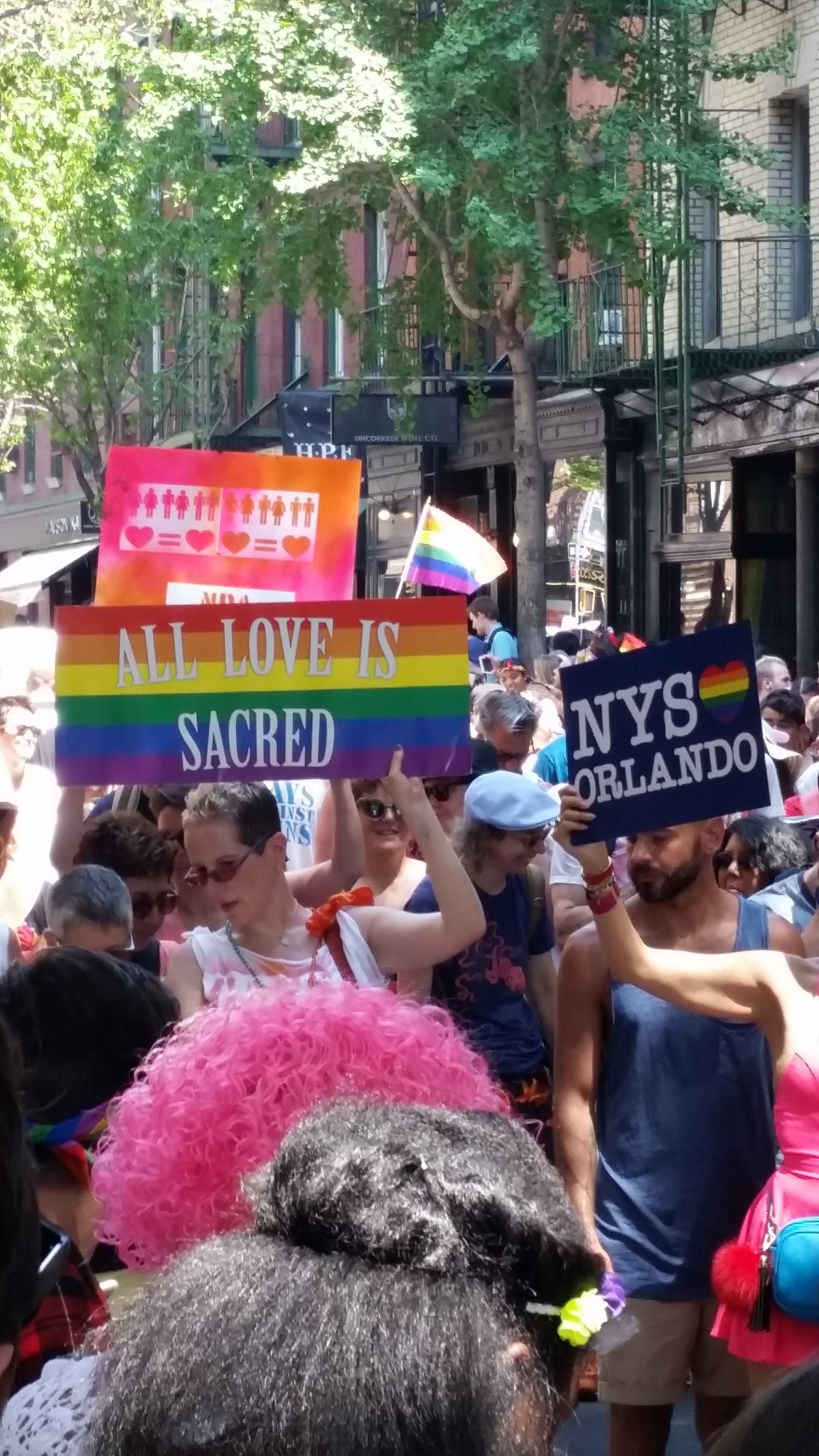The photograph captures a lively street scene, likely in New York, characterized by a densely packed crowd of people celebrating a gay pride parade. The participants, some sporting vibrant wigs and colored hair, brandish an array of signs and flags. Notable signs include a rainbow-colored one emblazoned with "All Love is Sacred" and another declaring "NYS Orlando" with a colorful heart. The crowd fills the lower part of the image, with some individuals facing the camera while others look away. The backdrop features older brick and stone buildings, indicative of New York's architectural style, adorned with wrought iron fences and interspersed with trees. The scene is colorful and chaotic, set in the middle of the day, with hues ranging from black, white, and brown to pink, light blue, dark blue, red, orange, yellow, green, blue, purple, and more, highlighting the vibrant and inclusive atmosphere of the event.